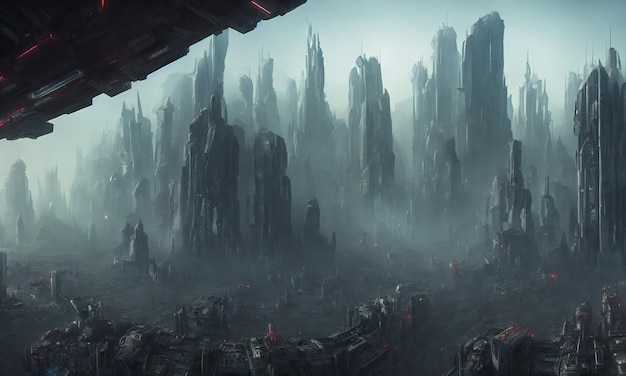This digital art piece depicts an eerie, post-apocalyptic sci-fi cityscape viewed from a high vantage point, likely a spacecraft. The background is filled with thick smog and a dull, overcast sky, infusing the scene with a sense of desolation and decay. The buildings, tall and jagged, resemble futuristic skyscrapers but are worn and dirty, almost appearing like spacecraft themselves, surrounded by a haze of pollution. Scattered pink lights can be seen punctuating the otherwise gray and dreary palette, adding a subtle glow to the scene. The foreground features a variety of smaller, grimy structures, contributing to the setting's overall rundown appearance. In the top left corner, some black and red spacecraft machinery partially blocks the view, hinting at the viewer's perspective from within a vessel. The combination of these elements creates a detailed and grim portrait of a dystopian world, blending high-tech architecture with a sense of abandonment and decay.